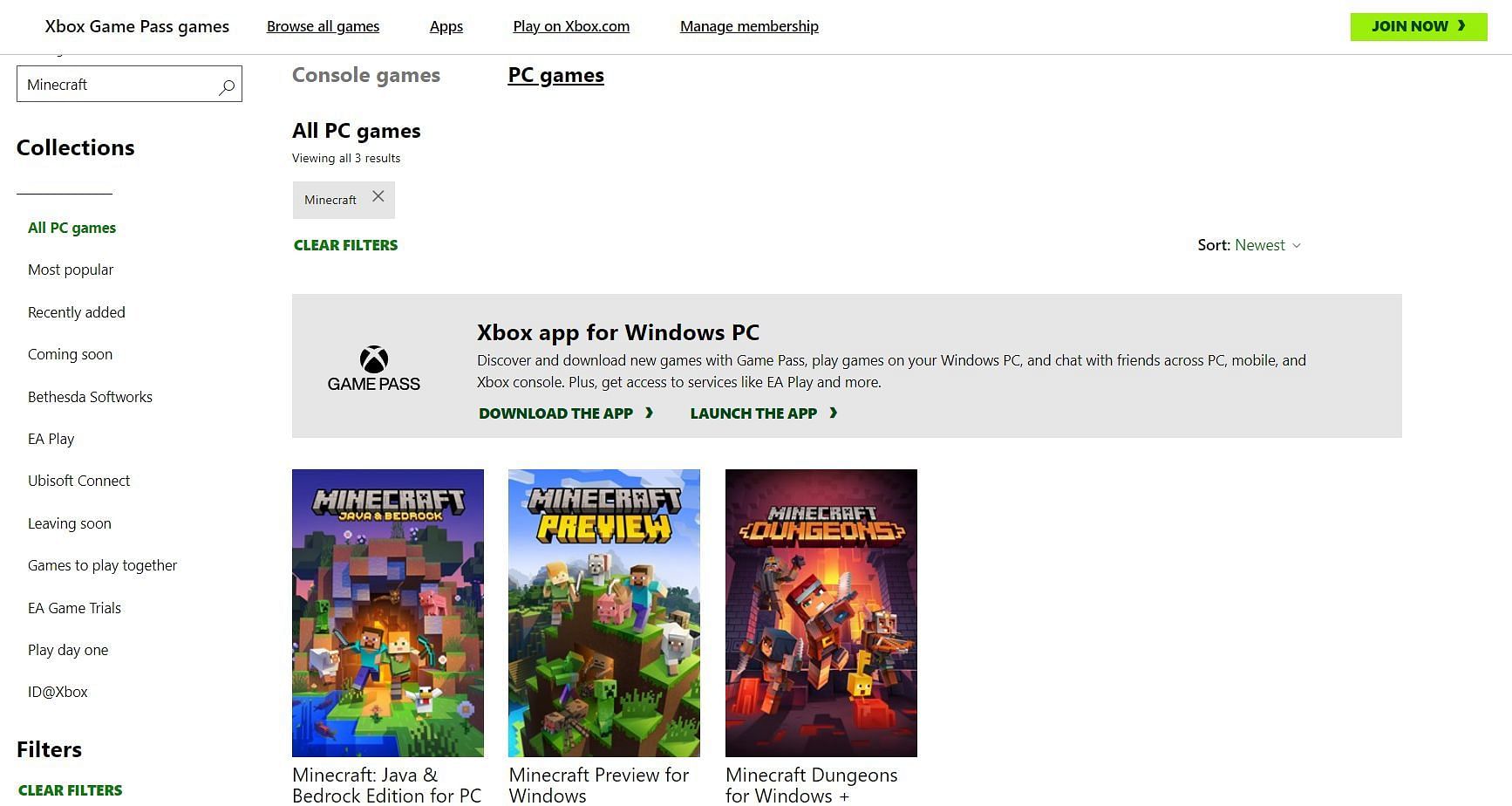This landscape-oriented screenshot captures the Xbox Game Pass interface, showcasing a variety of game offerings. In the upper right-hand corner, a light green "Join Now" button invites users to subscribe. The upper left corner prominently displays the heading "Xbox Game Pass Games," accompanied by navigational categories such as "Browse All Games," "Apps," "Play on Xbox.com," and "Manage Membership."

The layout is divided into two main columns. The left column, likely a sidebar, begins with a search bar where "Minecraft" is typed in. Below this, a bold title "Collections" designs the sorting categories: "All PC Games" (highlighted in green), "Most Popular," "Recently Added," "Coming Soon," "Bethesda Softworks," "EA Play," "Ubisoft," "Kinect," "Leaving Soon," "Games to Play Together," "EA Game Trials," "Play Day 1," "ID@Xbox." At the bottom of this section, bold headers "Filters" and "Clear Filters" (in green) offer additional sorting options.

The right section of the screen, corresponding with the highlighted "All PC Games" collection on the left, displays the search results for Minecraft. There are three visible results: "Minecraft Java & Bedrock Edition for PC," "Minecraft Preview for Windows," and "Minecraft Dungeons for Windows Plus."